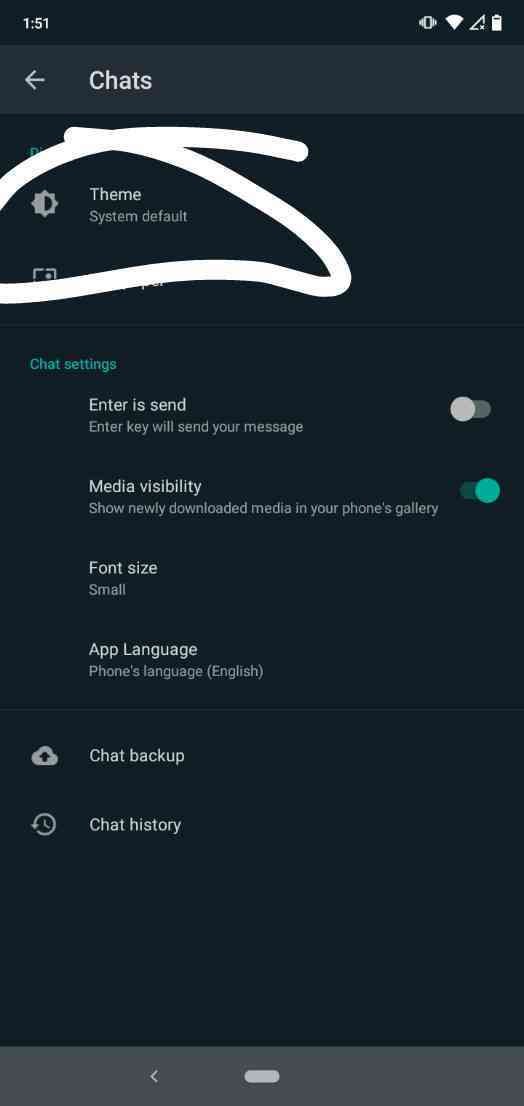Here is a detailed caption:

"In this image, a chat settings screen from a cell phone is displayed. At the top left corner, the time is shown, while the top right corner features icons for Wi-Fi connection, cellular signal strength, and battery percentage. Below the top status bar, the screen title 'Chats' is visible. Directly below, a white highlighted circle emphasizes the 'Theme' option. Subsequent to this are the 'Chat Settings' heading and four options: 'Enter is Send,' 'Media Visibility,' 'Font Size,' and 'App Language.' Among these, 'Media Visibility' is toggled on, indicated by a green circle, while 'Enter is Send' is not activated. Further down, there are options for 'Chat Backup' and 'Chat History.' The entire screen is set against a sleek black background. At the very bottom of the screen, there is a gray background strip with a small line centered at the bottom."